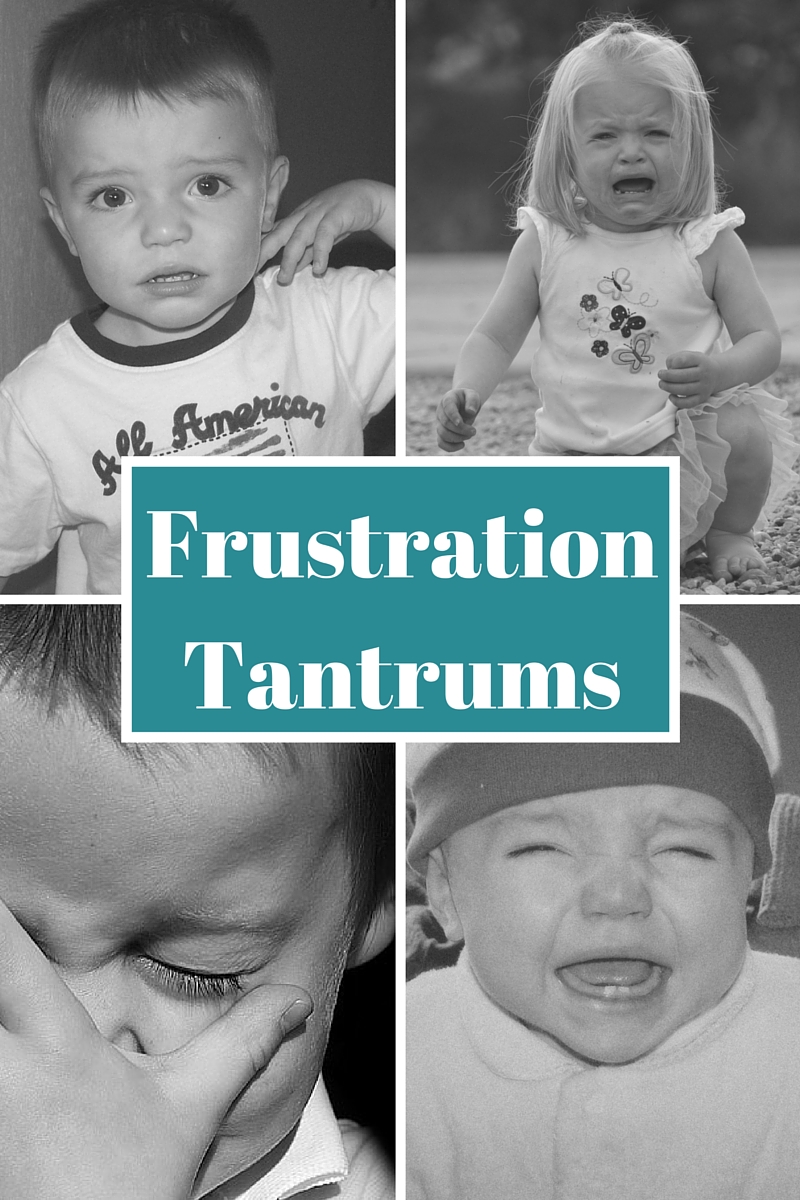The black and white image is arranged in a rectangular grid of four photographs, bordered by white lines, with the center featuring a teal rectangular background and white bold text stating "Frustration Tantrums." In the upper left photo, a small, light-haired Caucasian boy with large eyes is wearing a white t-shirt labeled "All American." His hand is near his ear, conveying his distress. The upper right photo depicts a young blonde girl, sitting outdoors in the dirt with her hands placed beside her. She is dressed in a white dress adorned with butterflies, crying with her mouth wide open. The bottom left image captures a close-up of a dark-haired boy with his eyes closed and one hand covering part of his face, clearly in distress. Finally, the bottom right photo shows another crying child wearing a knitted cap and a light-colored cotton outfit, though the child's gender is indeterminate. The collective imagery emphasizes the theme of emotional distress and frustration in young children.